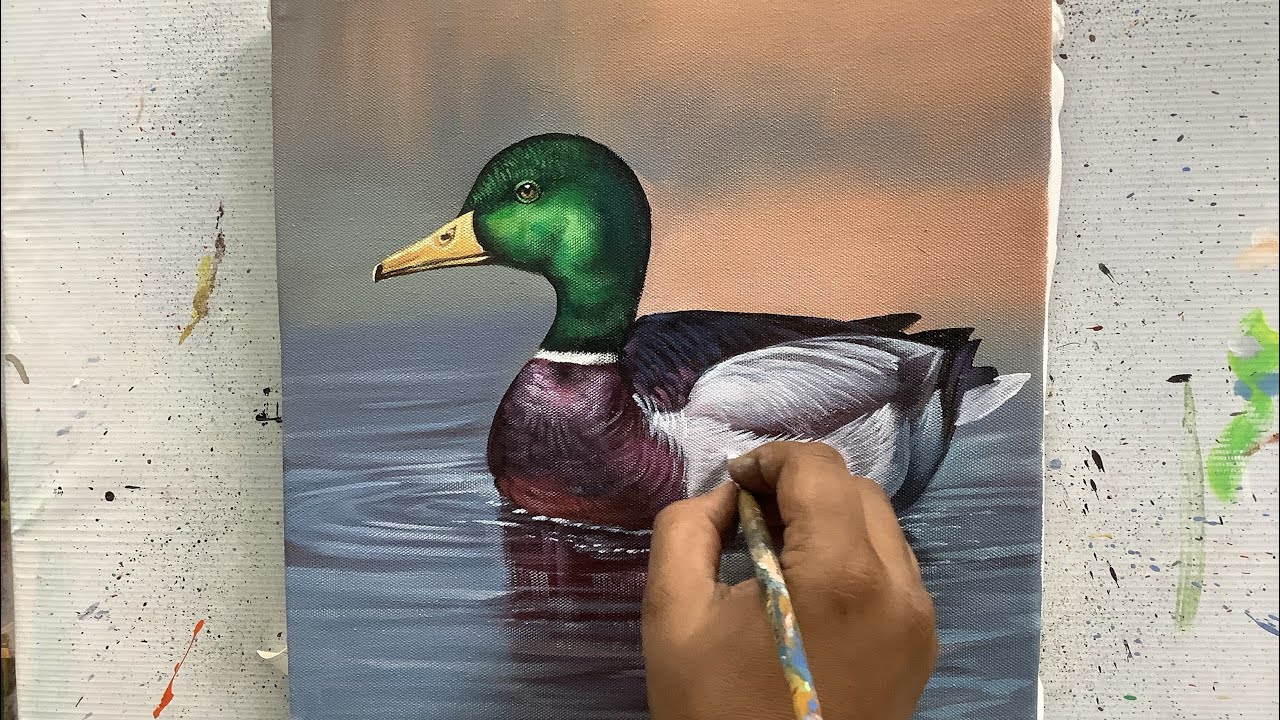In this detailed image, we see an artist, with tan hands speckled with paint, diligently working on a painting. The focal point is a realistic side profile of a mallard duck, characterized by its vivid green head, orange beak, small brown eye, and white ring around its neck. The duck's chest and back are depicted in a shiny brown hue, while its wing and side are white. The artist is using a well-worn paintbrush to apply details to the white area of the duck's body, which is floating serenely on water that features movement rings around it. The painting captures a tranquil scene with a backdrop of blue and orange sky reflecting on the water. The artist's workspace is cluttered with splatters of various paint colors, indicative of a surface that has seen many creative endeavors. The white flat surface on which the canvas rests is splotchy and covered in paint, emphasizing the artistic process behind the meticulous and skillful depiction.